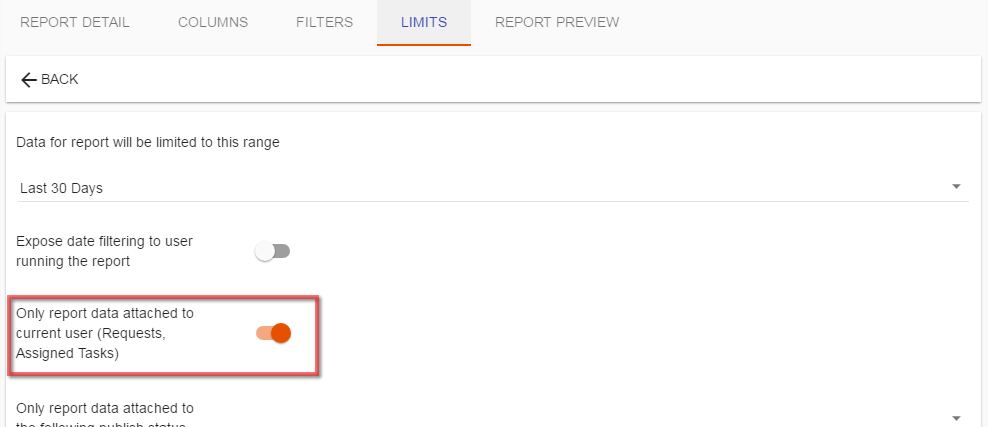This image depicts a web page interface primarily featuring a predominantly white background. At the top, there is a light gray rectangular banner with dark gray text. This banner comprises several clickable buttons, each labeled in all caps. The first label reads "REPORT DETAIL," followed by "COLUMNS," "FILTERS," and "LIMITS," with "LIMITS" being selected. The "LIMITS" button is darker gray due to its active selection and is underlined in red. The text for "LIMITS" has changed from dark gray to blue, indicating its active status. To the right, the text reverts to dark gray on a light gray background, labeled "REPORT OVERVIEW."

Beneath this banner, there is another white rectangular section featuring a bold black arrow and bold black text in all caps that reads "BACK." Below this, there is a section in a light gray-white gradient, containing black text that states, "Data for report will be limited to this range." This section shows "Last 30 days" with a dropdown menu on the far right, implying that different time ranges, such as a day or an hour, can be selected.

Further down, a new section is labeled, "Expose data filter to user running the report." It features a slider that is turned off, represented by a gray circle and a black background on the right side of the slider.

Another section follows, accented by a thick red border. It includes black text stating, "Only report data attached to the current user (request, assign task)." This section also contains a slider, positioned on the right-hand side and turned on. The background of the slider area is light gray with a light red background, and the circle on the right-hand side is red. Part of the text is cut off, but the visible portion includes, "Only report data attached to," followed by an incomplete sentence.